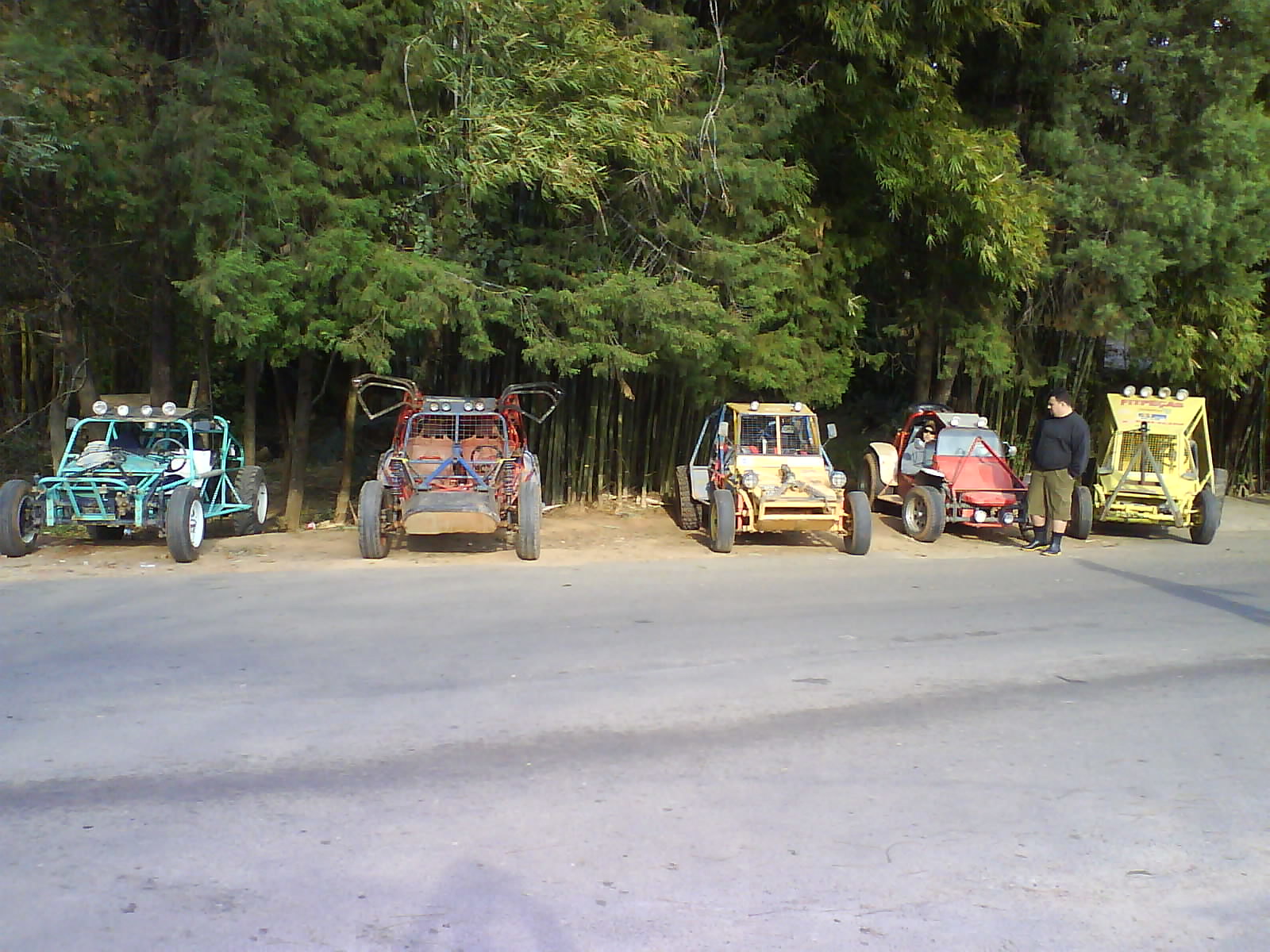The photograph features a lineup of five off-road dune buggies parked on the side of a wide, dusty paved road, which appears to be in a desert-like area. The background showcases a dense grove of tall, thick trees that form a nearly impenetrable barrier. From left to right, the buggies are positioned head-on, making their details clearly visible.

The first buggy on the left is a light blue or turquoise two-seater with a roll cage and roof-mounted off-road lights. Next to it is a red two-seater with distinctive suicide doors and four roof-mounted headlights. Adjacent to that is a yellow buggy with a squared nose and two headlights on both the hood and roof, reminiscent of a Volkswagen Beetle in design. The fourth buggy is red with two headlights on the bumper and two on the roof, with a passenger seated inside, wearing a cap and sunglasses. A man dressed in a long-sleeved black shirt, green capri pants, and black shoes stands in front of this red buggy, looking either at the passenger or the buggy next to it. The buggy on the far right is another yellow one, taller than the others, with four roof-mounted headlights and some indecipherable words on the windshield.

Overall, the image captures the rugged appeal and variety of these off-road vehicles against a backdrop of natural greenery and a dusty desert road.